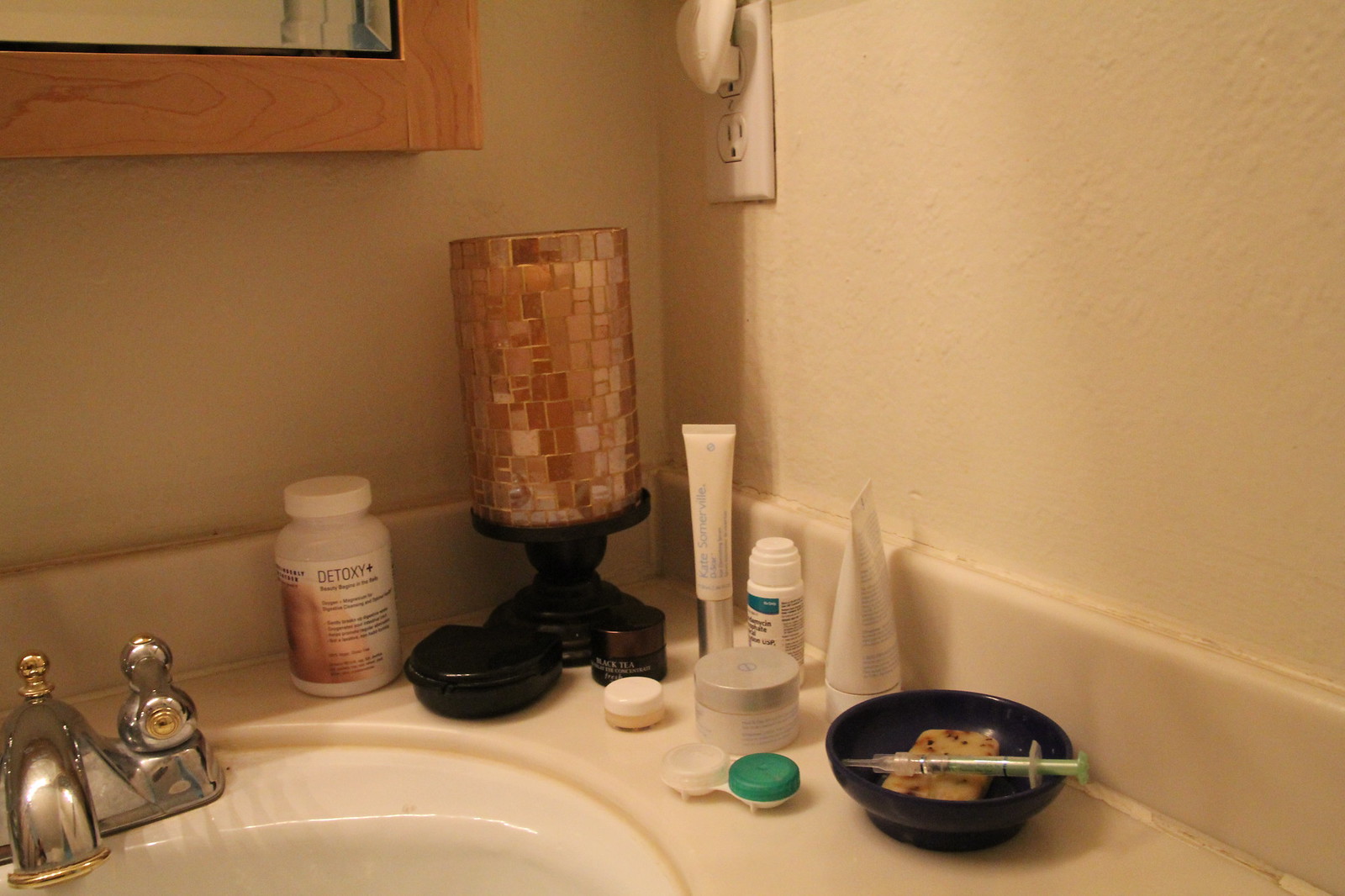This close-up photo captures the right side of a bathroom vanity sink countertop. The image highlights various objects arranged on the dark countertop set against an off-white wall. At the top left edge, a wooden-trimmed vanity mirror is partially visible. On the upper right section of the wall, there's a white electrical outlet with a white air freshener plugged in.

On the countertop, positioned at the corner, is a tall candle with a stained-glass design in assorted shades of brown, held in a black candle holder. To the left of the candle sits a white pill bottle, and in front of the candle, there's a black retainer holder.

A contact lens case, featuring a white and a green cap designated for the left and right eyes respectively, is also present. To the bottom right, a black bowl contains a needle or syringe alongside another unidentified object. Surrounding the candle are several different tubes. The silver stainless steel faucet with gold trim around the spout and pull tab is also visible, completing the setting.